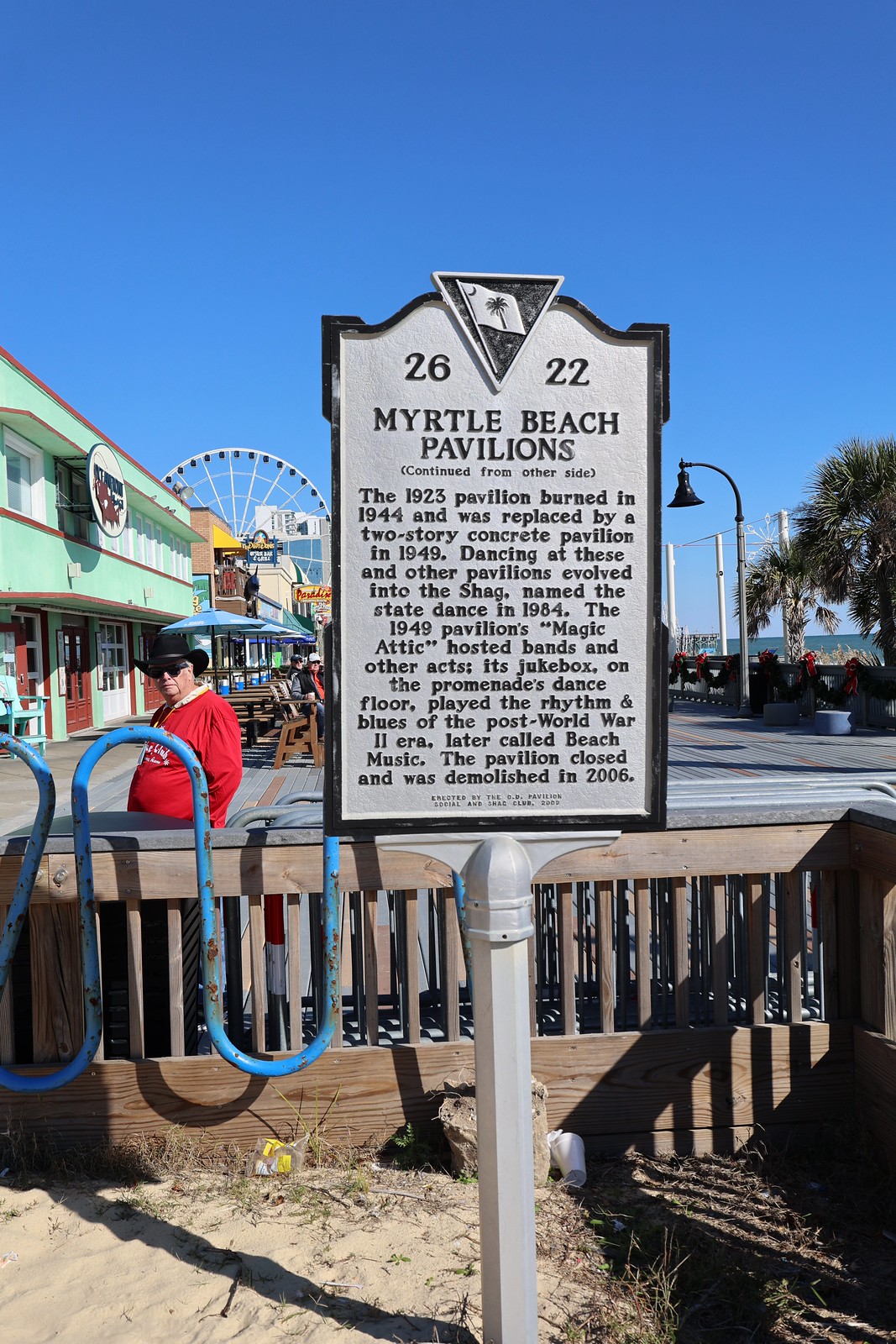The image showcases a historical marker prominently situated in a sandy surface at Myrtle Beach. The white marker with black text is centrally positioned in the frame. It reads at the top "2622" with a triangle between the numbers, pointing downward and featuring the South Carolina flag. Below, the sign commemorates the Myrtle Beach Pavilions and provides a rich historical narrative: the original 1923 pavilion, which burned down in 1944, was replaced by a two-story concrete pavilion in 1949. This pavilion's Magic Attic hosted bands and other acts, and its jukebox on the promenade's dance floor played rhythm and blues, which later became known as beach music. Dancing at these pavilions evolved into the state dance, the shag, in 1984. The pavilion eventually closed and was demolished in 2006.

The background of the image features a clear, blue sky without any clouds, typical of a bright, sunny day at the boardwalk. A white Ferris wheel and several tropical palm trees add a festive atmosphere, while a two-story pistachio green building with brown trim, possibly a hotel, is visible on the left. A man in a red sweatshirt and cowboy hat stands behind a fence near the building. To the right of the marker, there is a bike rack. The overall setting appears to be an outdoor recreational area, bustling with nostalgic landmarks and activities, capturing the essence of Myrtle Beach's historical and cultural heritage.